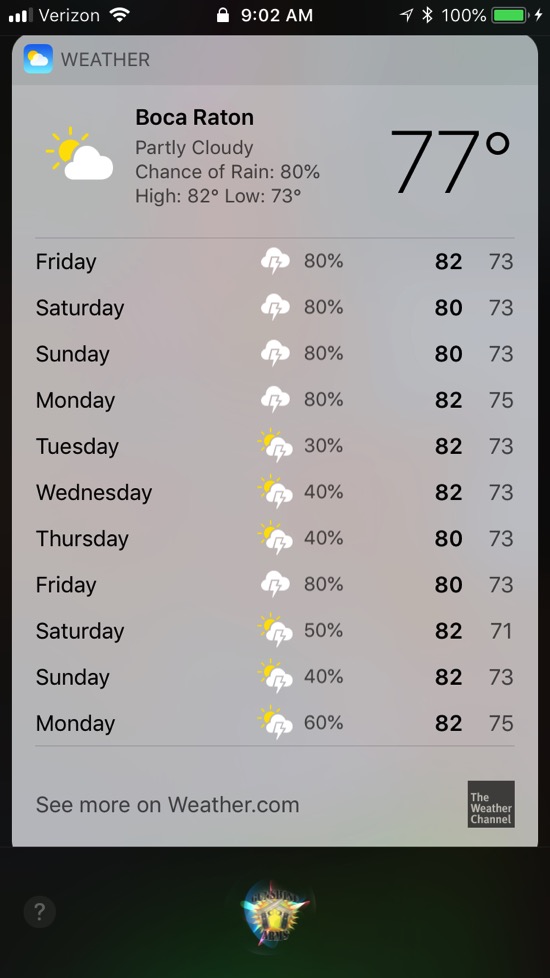This is a detailed screenshot of a smartphone's display showing various status icons and a weather forecast for Boca Raton. At the top, the phone has three out of four bars of Verizon cellular coverage, full Wi-Fi connectivity, a white padlock indicating a secure connection, the Bluetooth icon, a battery level at 100 percent, and the time displayed as 9:02 AM. 

The weather section reveals it is currently partly cloudy in Boca Raton with an 80 percent chance of rain. The present temperature is 77°F, with forecast highs and lows of 82°F and 73°F respectively. The upcoming week's forecast predominantly predicts thunderstorms with an 80 percent chance on Friday, Saturday, Sunday, and Monday. The highs are consistently around 80°F, and the lows around 73°F. The forecast shows a slight chance of thunderstorms on Tuesday at 30 percent, increasing to 40 percent on Wednesday and Thursday. Thunderstorm chances spike to 80 percent the following Friday, then drop to 50 percent on Saturday, and 40 percent next Sunday, with Monday showing a 60 percent chance.

At the bottom right corner of the screen is a box labeled "The Weather Channel," and the the forecast suggests checking weather.com for more detailed information.